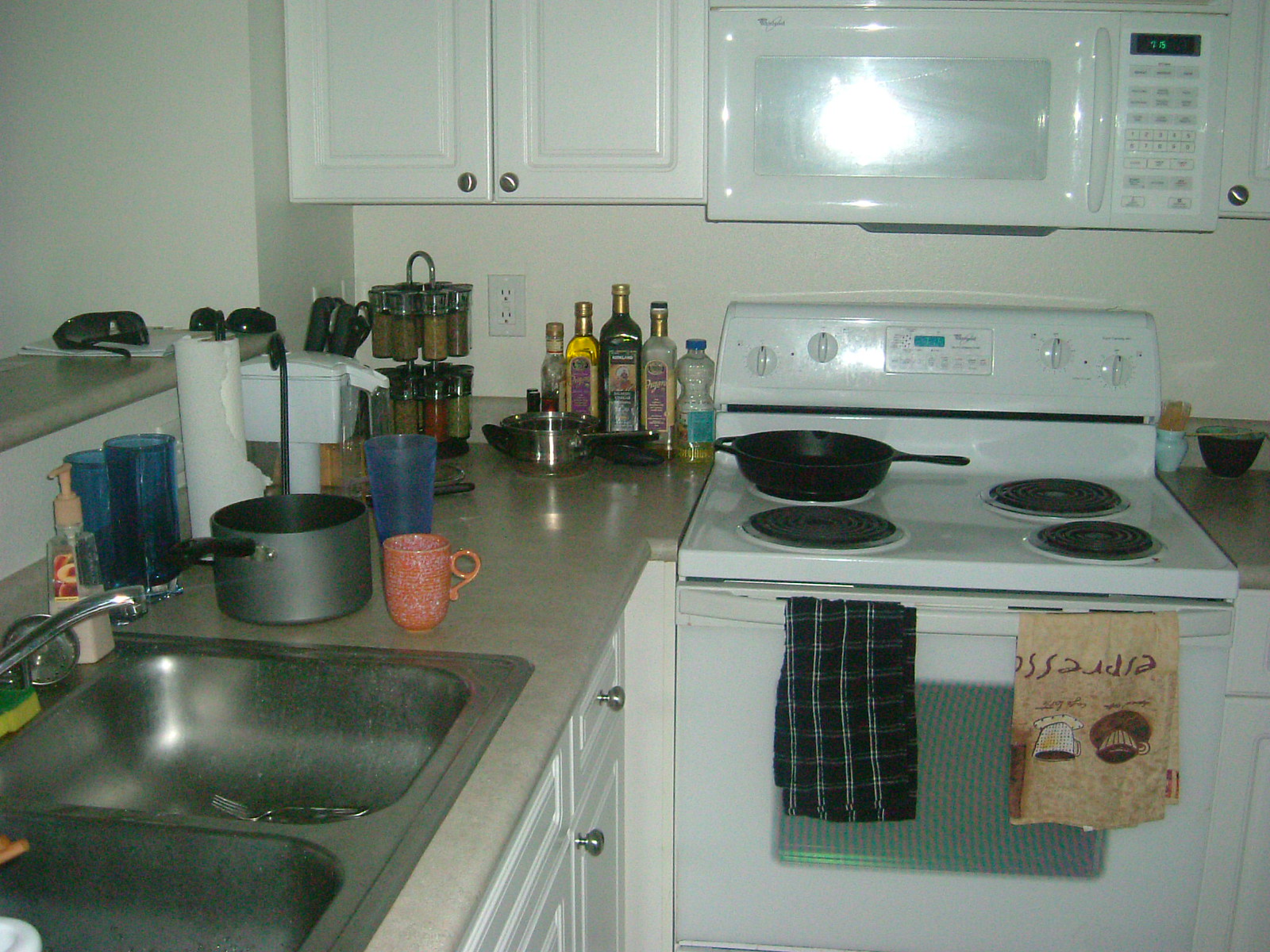In this detailed kitchen snapshot, the camera captures a familiar domestic scene centered around a double sink and stove. To the left, a stainless steel double sink is equipped with a classic faucet and a nearby sink stopper. Resting on the sink edge is a green and yellow sponge, paired with a clear soap pump reminiscent of those sold at Bath and Body Works, suggesting this image might be from around 20 years ago. The surrounding countertop, a light gray laminate, hosts a variety of everyday items. In the corner, a spice rack stands beside bottles of oil, and there are several pots scattered nearby. A paper towel holder is also visible. 

Adding a pop of color, a blue plastic cup sits empty, juxtaposed with an orange coffee cup adorned with white speckles. Directly in front of us, the electric stove is adorned with two kitchen towels draped over the oven handle—one in a black and white checkered pattern, the other featuring an espresso design with two coffee cups on a brown background. A black cast-iron skillet rests on the stovetop, completing this snapshot of a well-used, functional kitchen.